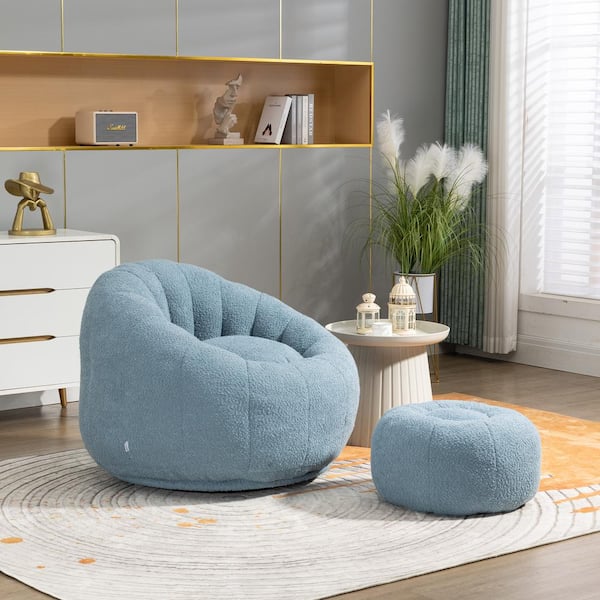The photograph captures a cozy and stylish room featuring a distinctive light blue chair and matching footstool, both resembling bean bags but with a segmented, fruit-like design and a soft, fuzzy exterior. These comfortable pieces rest on a large white rug with orange splatters and closely-set gray rings, reminiscent of tree rings. To the left of the chair, a small circular bench displays some ornamental figurines. The background showcases a sleek, grey wall adorned with gold vertical stripes and an inlaid shelf bordered in gold. The shelf houses a radio-like device, a ‘shushing’ face sculpture, and a stack of five books. Below it sits a white lacquer chest of drawers with rounded edges and gold handles, topped by a metal sculpture depicting a head resting on hands, wearing a hat. To the right, a white pot stand holds a green plant with unique feather-like flowers. The scene is completed by tall blue and white curtains framing a right-side window with white plantation shutters, allowing sunlight to stream into the room.